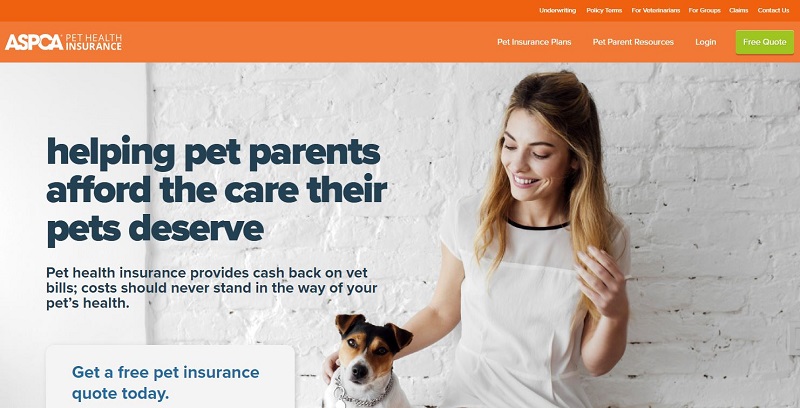**Website Description for ASPCA:**

The ASPCA website features a top navigation bar in dark orange with a lighter orange strip beneath it. Though the text on the dark orange bar is too small to read, it is likely intended for utility links or navigation aids. Just below this, "ASPCA" is prominently displayed, ensuring brand recognition.

The focal point of the page is an emotive image of a woman, dressed entirely in white, except for a black stripe that accents the area around her top teeth. She has long blonde hair and is seen tenderly looking down at her dog, who is a Jack Russell Terrier mix. The setting is a brick wall painted white, which provides a clean backdrop.

The dog has a characteristically small, white body with a black nose, brown markings around its eyes, and additional black markings. The dog's ears feature a distinct black coloration with brown trimming. The attentive dog is looking directly at the camera, wearing a silver, constricting collar designed to tighten when pulled.

Accompanying the image, the caption reads: "Helping pet parents afford the care their pets deserve. Pet health insurance provides cash back on vet bills. Costs should never stand in the way of your pet's health." This message underscores the ASPCA's mission to ensure pets receive necessary care by making pet health insurance accessible.